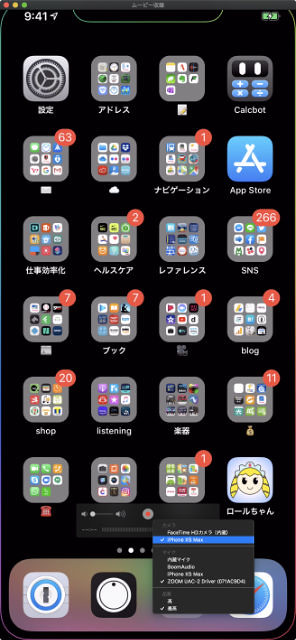A detailed screen capture of a smartphone interface featuring a black background. The display shows a grid of 20 square app icons arranged in four columns and five rows. Several icons feature an orange oval in the upper right corner, each containing a number, indicating notifications. The bottom of the screen includes a rectangular dock with additional apps. Notable features include a circular camera icon and, to its left, a white square with a circle and a power symbol. The app icons vary in appearance; some contain Asian characters, while others are labeled in English. The time displayed in the upper right corner is 9:41. Many app icons also display smaller square grids with three columns and three rows. In the lower right corner, there is an app featuring a cartoon face of a character with long blonde hair. Visible apps include the Apple Store, SNS, Blog, Listening, Shop, and Calcbot. This image is either a computer-generated mockup or an actual screen capture.